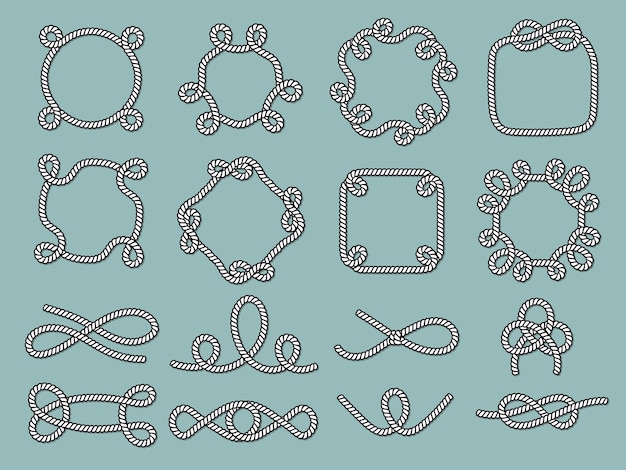The image is a digitally created composition showcasing various hand-drawn rope designs against a greenish-blue, almost turquoise background. The design is laid out in a grid, featuring four rows and four columns of these rope illustrations, making a 4x4 pattern. 

**First Row**: The top-left corner starts with an oval rope design with curls on each corner. Next to it is a rounded hexagon-like shape, adorned with small circles at its vertices. The third one is a rounded square with multiple small circles along its edge. The row concludes with a square design featuring a figure-eight knot at the top.

**Second Row**: This row begins with a blade-shaped rope design with circular forms at the edges. Following that is a diamond shape with figure-eight knots on each corner. The third design is another rounded square, but this time with small interior circles at each corner. The row ends with an octagonal shape filled with curved lines or circles.

**Third Row**: Here, the focus shifts more to knots rather than frames. The first design shows a simple figure-eight knot. This is followed by a design consisting of three ovals, with one large oval in the center flanked by smaller ones. The third design evokes the shape of a noose, featuring a central loop with two thinner rope lines extending outward. The row concludes with a three-leaf clover-like shape.

**Fourth Row**: The bottom left begins with a pretzel-like shape, while the next design to the right features an eye-shaped outline with two small circles inside. The third from the left is a W-shaped rope with a central circle. The final design in the bottom right corner showcases another figure-eight knot.

These detailed and varied rope illustrations seem more artistic and possibly educational, illustrating different types of knots and rope arrangements. The use of white and black lines to represent the twists of the rope against the monochromatic greenish-blue background adds a visual and instructional aesthetic to the image.